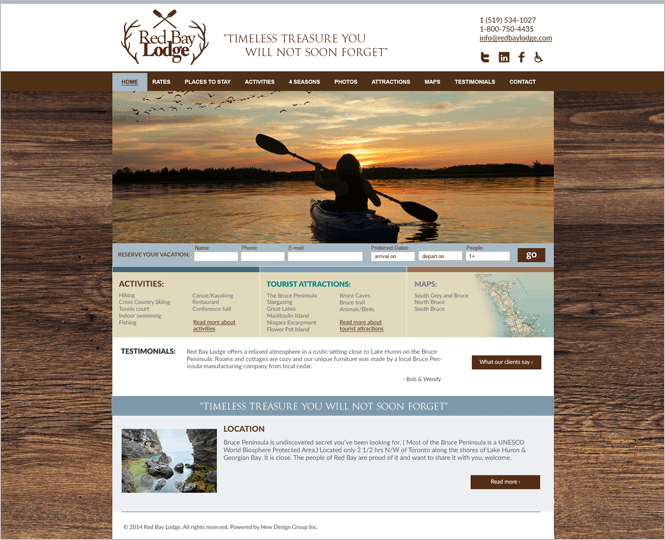The image displays a website for Red Bay Lodge with a well-organized and visually appealing layout. At the top, there is a prominent white section. Centrally placed, two decorative branches adorned with paddles frame the lodge's name "Red Bay Lodge" written in a rustic brown font. Accompanying this, to the right, is the lodge’s tagline: "Timeless Treasure You Will Not Soon Forget". Further right, contact information is provided, including two phone numbers and an email address: information@redbaylodge.com. Social media icons for Twitter, Instagram, and Facebook are conveniently located nearby, along with an icon indicating the website’s accessibility features.

Beneath this header, there's a wooden-textured background enhancing the lodge's rustic charm. A captivating photograph of a person canoeing at sunset over serene waters graces the top section, setting a tranquil and inviting scene. Navigation tabs are neatly arranged at the top, allowing easy access to pages such as Home, Rates, Places to Stay, Activities, Four Seasons, Photos, Attractions, Maps, Testimonials, and Contact. The Home tab is currently active.

Below the main image, there is a call-to-action section titled "Reserve Your Vacation", where visitors can input their name, phone number, email, and preferred dates for their stay. This section is highlighted by a framing background contrasted with earth-toned colors.

Further down, a brown section provides information about activities and tourist attractions, followed by a white area featuring testimonials. A brown button prompts users to read what clients have to say. At the very bottom of the page, details about the lodge's location are presented, along with another brown button labeled "Read More". Overall, the website combines functionality and aesthetic appeal to create an inviting and informative experience for prospective guests.